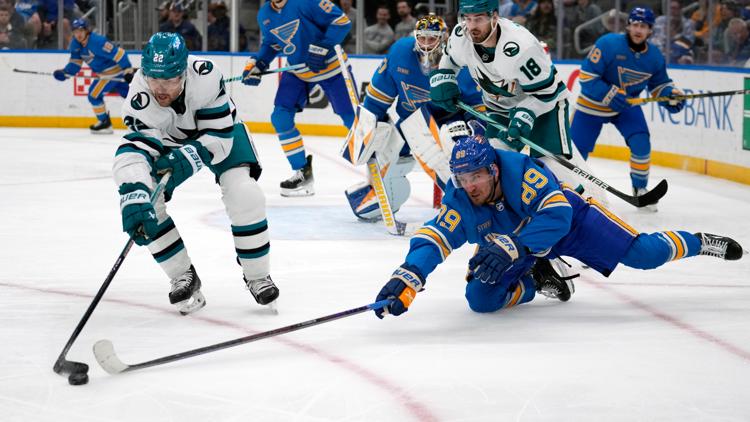The action-packed scene on the indoor ice rink captures a thrilling moment in a hockey game between two teams. The team in bright blue uniforms with yellow accents is clashing intensely with their opponents, who don white jerseys accented with hunter green. The tension heightens as a player in the blue team scrambles on his knees, desperately fighting for control of the black puck against an opposing player in white and teal, who stands resolutely. Among the players, the blue team outnumbers their opponents five to two in this frame. The ice surface gleams white under the bright lights, crisscrossed by distinct red lines. In the background, the spectator stands are filled with eager fans, and the word "BANK" is visible on the right-hand side, adding to the vibrant atmosphere of the arena.